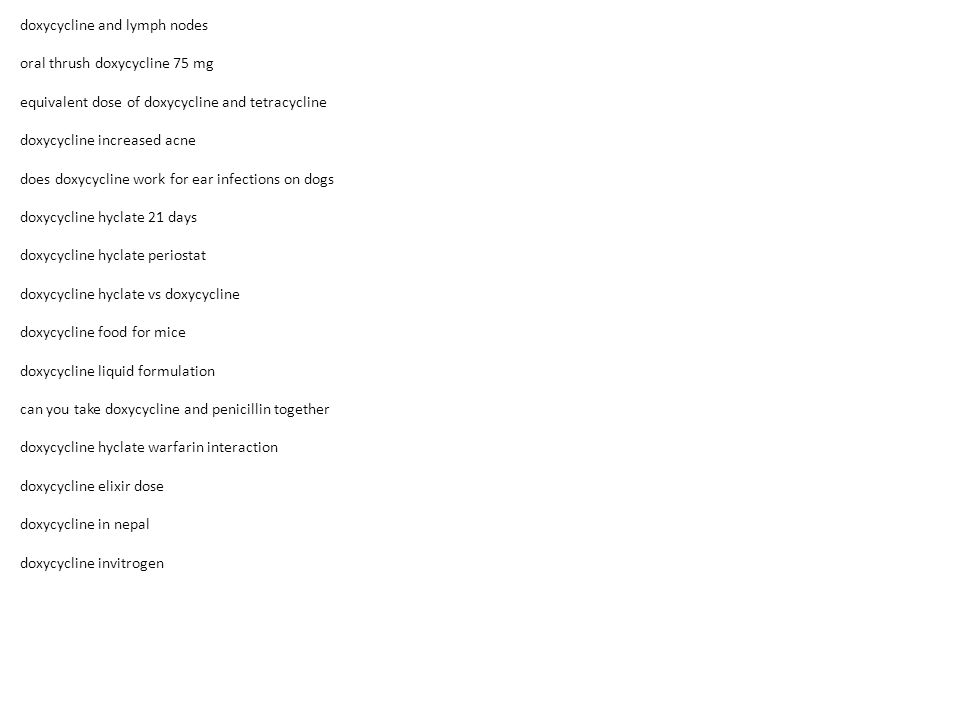The image features various doxycycline medications set against a white background. These include:

- Doxycycline 75 mg, used to treat conditions like acne.
- Information about doxycycline's use in managing ear infections in dogs.
- Details on prolonged doxycycline courses, such as high-dose treatment for 21 days.
- Comparisons between different doxycycline formulations, including Periostat.
- Insight into doxycycline's liquid formulations and dosages, such as elixirs.
- Notes on the concurrent use of doxycycline with other medications, including tetracycline, penicillin, and warfarin, highlighting potential interactions.
- Specialized doxycycline treatments, covering applications like nipple infections and its use in laboratory settings, such as for mice in vitrogen studies.